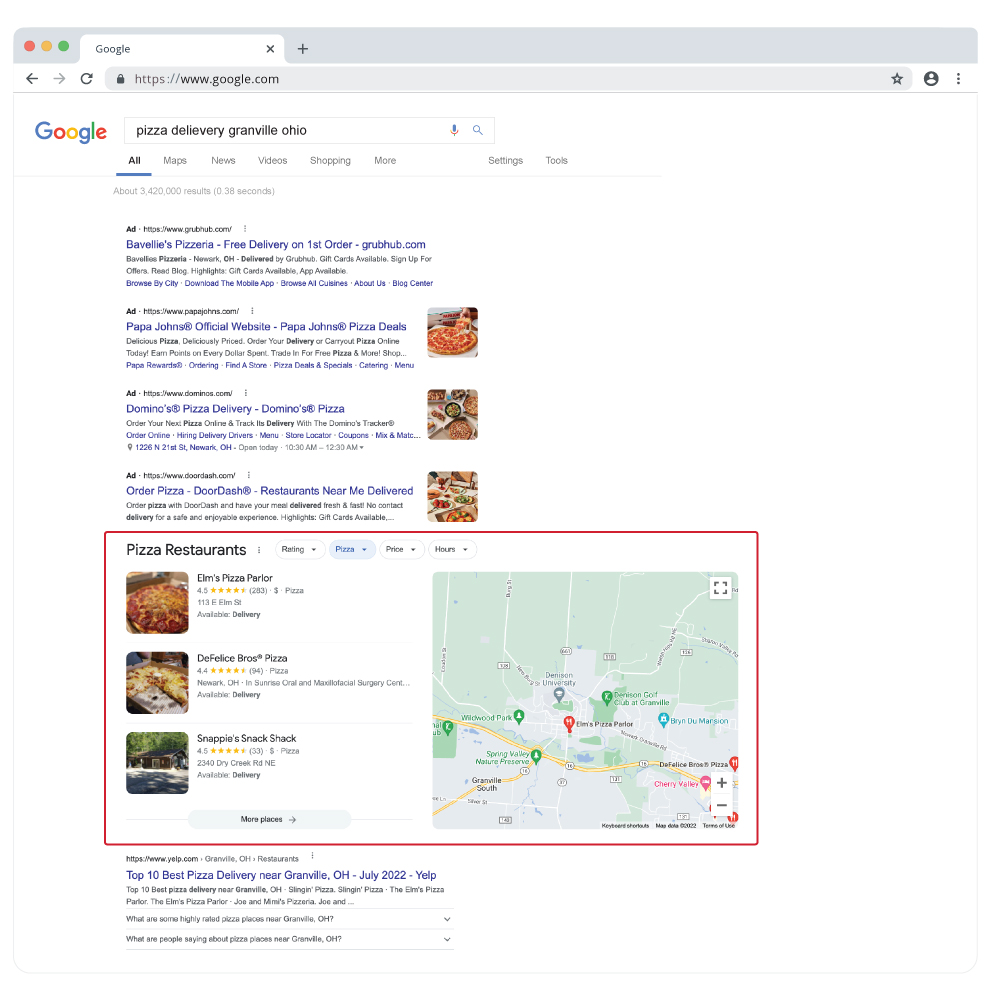The image depicts a Google search results page. The familiar Google logo is positioned in the top left-hand corner, indicating the authenticity of the page. In the search bar next to the logo, the phrase "pizza delivery in Granville, Ohio" has been entered. Below the search bar lies a navigation menu with clickable tabs labeled "All," "Maps," "News," "Videos," "Shopping," "More," "Settings," and "Tools," allowing the user to refine their search.

The first four search results are marked with the word "Ad" to differentiate them from organic results. Each of these ads is prominently displayed in blue lettering. The first ad reads "The Value’s Pizzeria – Free delivery on first order – grubhub.com." The second ad is titled "Papa John’s Official Website – Papa John’s Pizza Deals." The third advertises "Domino’s Pizza Delivery – Domino’s Pizza," while the fourth one states "Order Pizza – DoorDash – Restaurants Near Me Delivered." Beneath each of these blue-labeled ads are brief descriptions in black lettering, providing additional details about the offerings.

Below the advertisements, a large, horizontally-oriented rectangle bordered in red stands out. This section is headed with the title "Pizza Restaurants" in black lettering on the top left corner. It features tabs for filtering by "Rating," "Prices," and "Hours." Under this section, three specific pizza places are highlighted. "Elm’s Pizza Parlor" appears first, accompanied by a thumbnail image of a large pepperoni pizza, its rating, address, and delivery information. Next is "Feliz Bros Pizza," showcased with a thumbnail of another pizza, along with its ratings, location, and delivery details. The third listing is "Snappy Snack Shack," which features a thumbnail image, possibly of a house or restaurant, along with its ratings, address, and delivery information.

To the right of the search results, a small thumbnail map is displayed. This map includes pins marking the locations of the listed pizza restaurants, providing a visual representation of their whereabouts in Granville, Ohio.